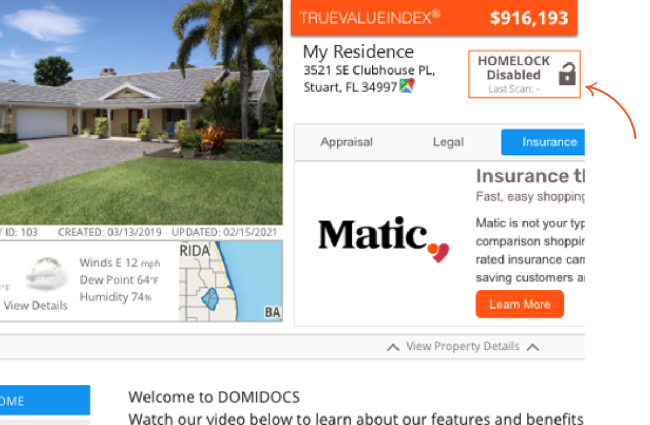Title: Comprehensive Overview of Property at 3521 S.E. Clubhouse, P.L. Stewart, Florida 34997

“True Value Index: 916,193 money. A detailed appraisal and insurance information display for the residence located at 3521 S.E. Clubhouse, P.L. Stewart, Florida 34997. The home lock is shown disabled, with the last scan revealing an unlock padlock, indicated by an orange arrow.

The highlighted sections emphasize various aspects: 'appraisal,' 'legal,' and 'insurance,' with 'insurance' highlighted in blue. A specific focus on ‘Insurance T’ denotes fast and easy shopping options. Additionally, the caption mentions, ‘Matic is not your type,’ suggesting alternative comparison shopping and rated insurance options via ‘Insurance Cam,’ aimed at saving customers money.

The image features a house with a well-maintained green grass yard. Property details include ID: 103, created on 03/13/2019, and updated on 02/15/2021. Current weather conditions at the location show winds from the east at 12 miles per hour, a dew point of 64, and humidity at 74%.

Further, the caption introduces ‘Domidox,’ inviting viewers to watch a video below to learn about the platform’s features and benefits. However, the benefits mentioned appear to be in Welsh: 'Yn ddiweddar, mae'r cyfrifiadau a'r cyfrifiadau yng Nghymru yn ymwneud â'r cyfrifiadau yng Nghymru.'”

This caption provides a comprehensive and detailed description of the property, its appraisal and insurance information, and additional platform details, making it informative for potential viewers or interested parties.